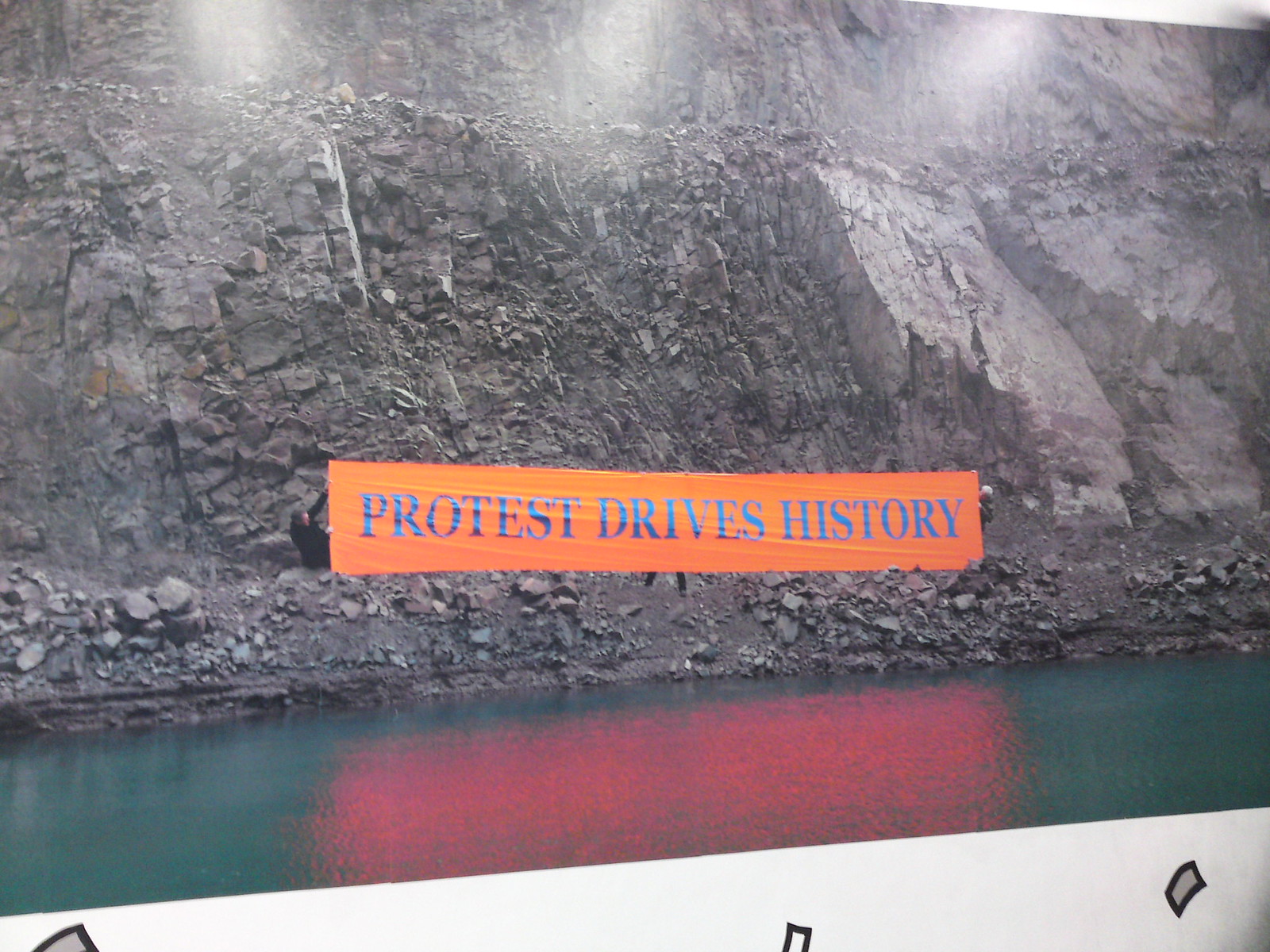The image is a full-color outdoor photograph depicting a dramatic rocky mountain cliff with varying shades of gray. The cliff dominates the background, featuring a mix of smooth and jagged rocks. At the foot of the cliff, there is a serene, greenish body of water, completely calm with no visible waves or ripples. Positioned at the center of the image and slightly elevated is an orange banner with bold blue text declaring "Protest Drives History" in capital letters. Three individuals are involved in holding the banner: one person is visible on each end, and a third person stands behind it, ensuring the banner is stretched taut. The time of day is indeterminate, but there are three lights at the top illuminating the rock face, suggesting additional lighting. In the foreground, what appears to be a wall partially frames the scene. This captivating image captures a peaceful protest set against a rugged, natural backdrop.